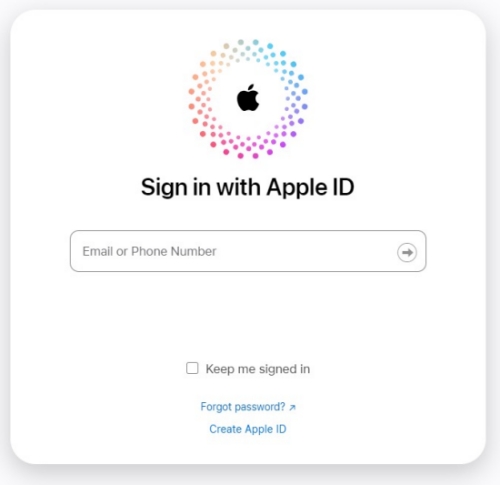This image is a web-based sign-in screen for an Apple ID. It features a white square with rounded corners, encompassed by a misty gray border. At the top center of the white square, there's the iconic Apple logo, above a multicolored, circular halo with dots in shades of blue, purple, pink, and yellow-orange, creating a vibrant visual accent.

Just below the halo, centrally positioned about a third down from the top, is the prompt "Sign in with Apple ID" in clear, bold text. Underneath this prompt is a horizontal gray text box labeled "email or phone number," used for inputting user credentials. To the right of this text box, there's a gray arrow within a circle, oriented to the right, indicating the direction to proceed.

Further below, after some empty space, is a small square checkbox accompanied by the text "Keep me signed in," allowing users to stay logged in across sessions. Finally, at the bottom of the sign-in interface, there are two small, blue, clickable links: "Forgot password" and "Create Apple ID," providing additional options for users who need to retrieve their password or create a new account.